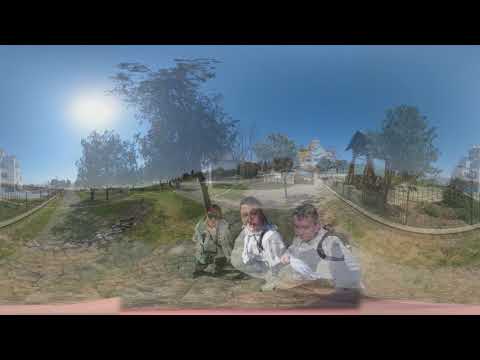The image appears to be a distorted, panoramic shot transitioning between two scenes, possibly a screen grab from a video. It takes place in an outdoor urban park featuring grassy areas, wooden structures, fences, and several trees. In the background, there are distant buildings, some with brown and white rooftops, adding to the urban setting. The sky is blue with a glaring, unfocused white sun, and there's a body of blue water visible on the right side. The foreground depicts three young people sitting on the ground; one is wearing a gray shirt, while the other two are in white shirts with black backpacks. They might be holding something as black bands appear over their left shoulders. The image is heavily distorted and foggy, making it difficult to discern details clearly, but a grayish basketball court with a hoop is noticeable behind the kids. The bottom and top of the image are marked by black lines, adding to the distortion and blur.